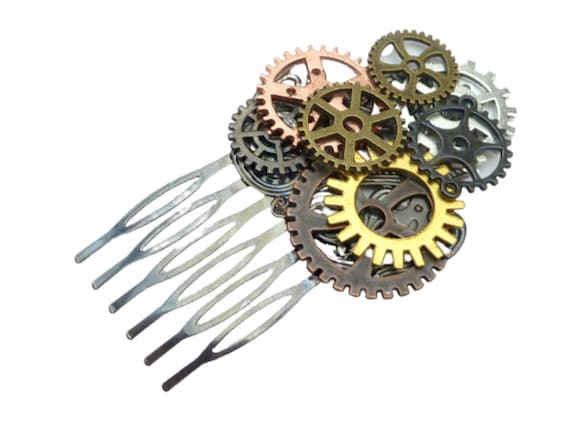This close-up product photo showcases a handmade barrette-style hair clip adorned with an intricate steampunk design. Nine metal gears in various shapes, sizes, and colors—including brass, gold, black, coppery, and silver—are meticulously arranged and stacked on top of one another. Some gears feature short knobs while others have elongated ones, and their centers vary from open spaces to intricate details with circles and lines. The clip also includes six elongated metal rods with small holes, positioned off to the left at an angle resembling 7 o'clock if viewed as a clock face. These rods add to the layered complexity of the design, contributing to the overall aesthetic. The careful craftsmanship ensures no visible glue, solidifying its handmade quality. With its visually striking appearance, this hair clip is perfect for completing a steampunk costume or enhancing a daily outfit that fits a unique, eclectic style.